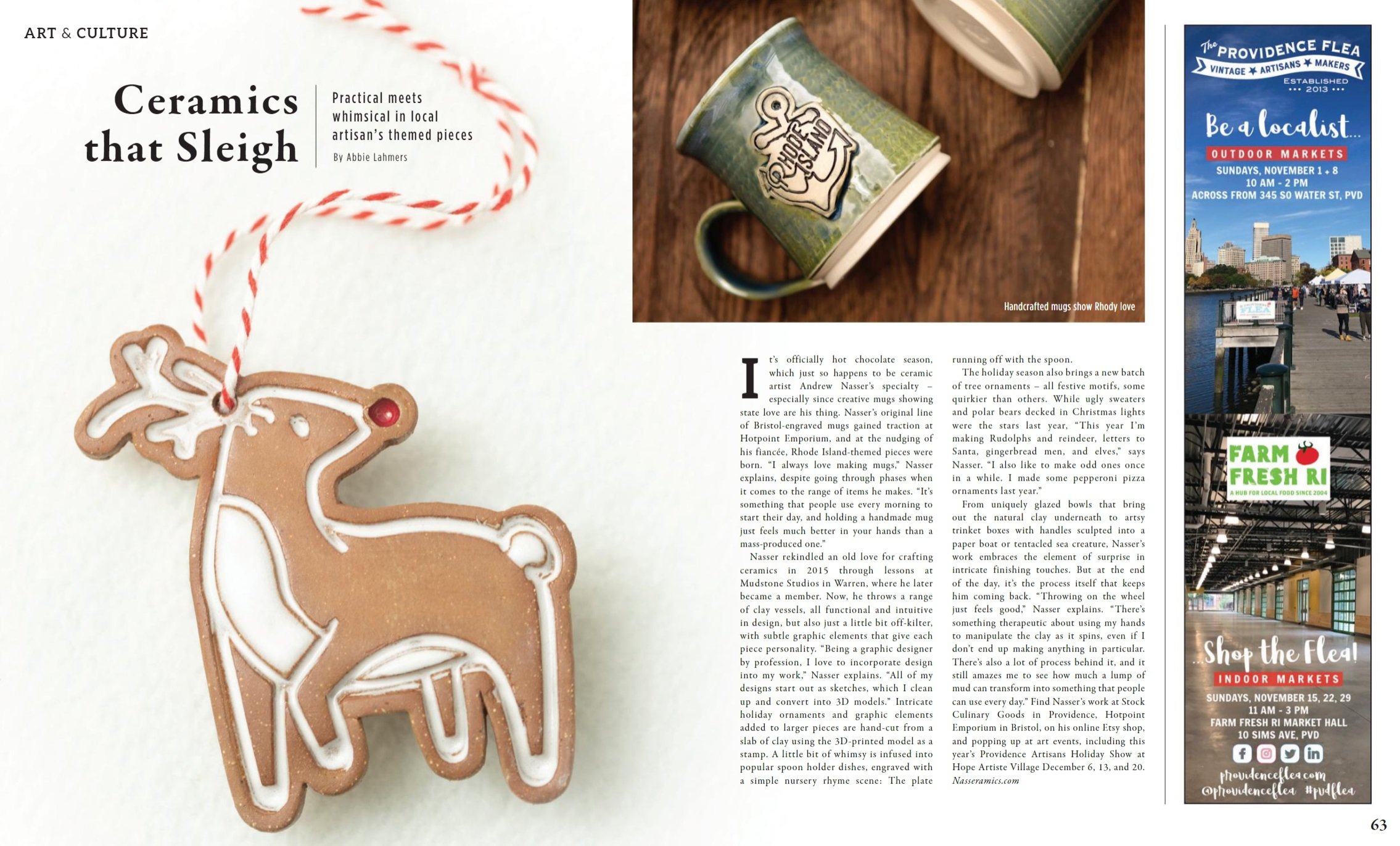This is a detailed page out of a magazine or a section of the Sunday newspaper with the heading "Art and Culture" in the upper left-hand corner. The main feature showcases a whimsical ceramic reindeer made by local artisan Abby Lahmers, with a red and white string laced through a hole, suggesting it could be worn as a necklace. The caption cleverly reads, "Ceramics that Slay,” combining practical use with whimsical design. 

The page also includes an image of two green mugs; one prominently displays the word “Rhode Island” superimposed over an anchor, while the other mug is partially visible. On the far right, there is an additional advertisement for a fresh farm or flea market, emphasizing the local and artisanal theme of the spread. The background of the upper section is white, contributing to the clean and inviting presentation of the art and culture pieces.